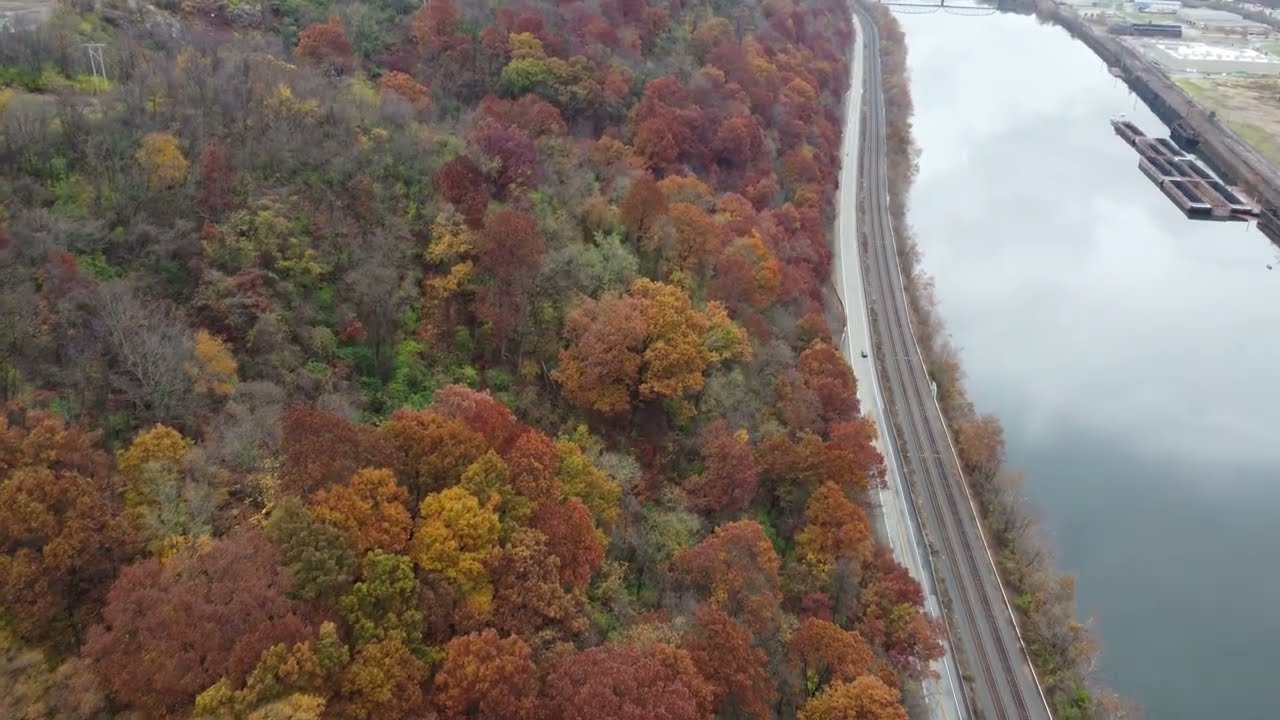This aerial photo, taken during the fall, provides an expansive view of vibrant autumn foliage. The image is horizontally oriented, with a vertically aligned roadway and train tracks running through its center, slightly skewed towards the right. On the left side of the road, the ground is densely covered with a forest of vividly colored trees—shades of green, yellow, orange, red, and purple, capturing the essence of autumn. The right side of the image features a serene river, its water reflecting a light blue sky, transitioning to a slightly more purple-gray hue towards the bottom right. The river extends from the top right to the bottom right corner, with some barges visible on its surface. Between the river and the train tracks lies a strip of bushes and low-lying trees. Beyond the river, there are fields and grassy areas interspersed with some low-lying buildings. This detailed scene is viewed from a high vantage point, reducing vehicles to mere dots on the roadway.